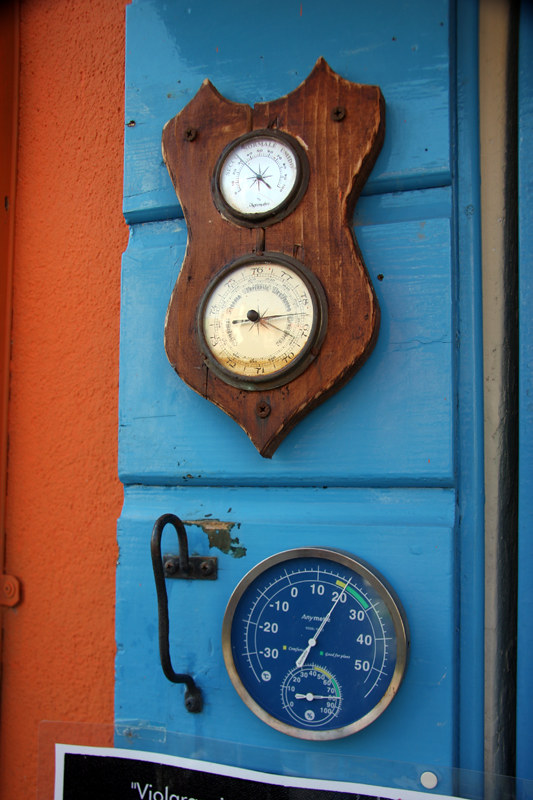Mounted on a wooden wall, a shield-like wooden plaque is secured with three large screws. This plaque displays three distinct gauges, possibly indicating various environmental or mechanical measurements. The top section features two gauges: a smaller one above and a larger one below, each with a single hand pointing to unknown metrics. Below these, there is a prominent circular gauge. This gauge has a scale ranging from -30 to 50, with a green zone spanning 20 to 30 and a yellow caution zone from 15 to 20. The needle currently points to 20, suggesting it is within the normal range. Within this circular gauge, there is an additional smaller gauge with a scale from 0 to 100, and its needle points to 80, which is situated at the upper end of the green zone.